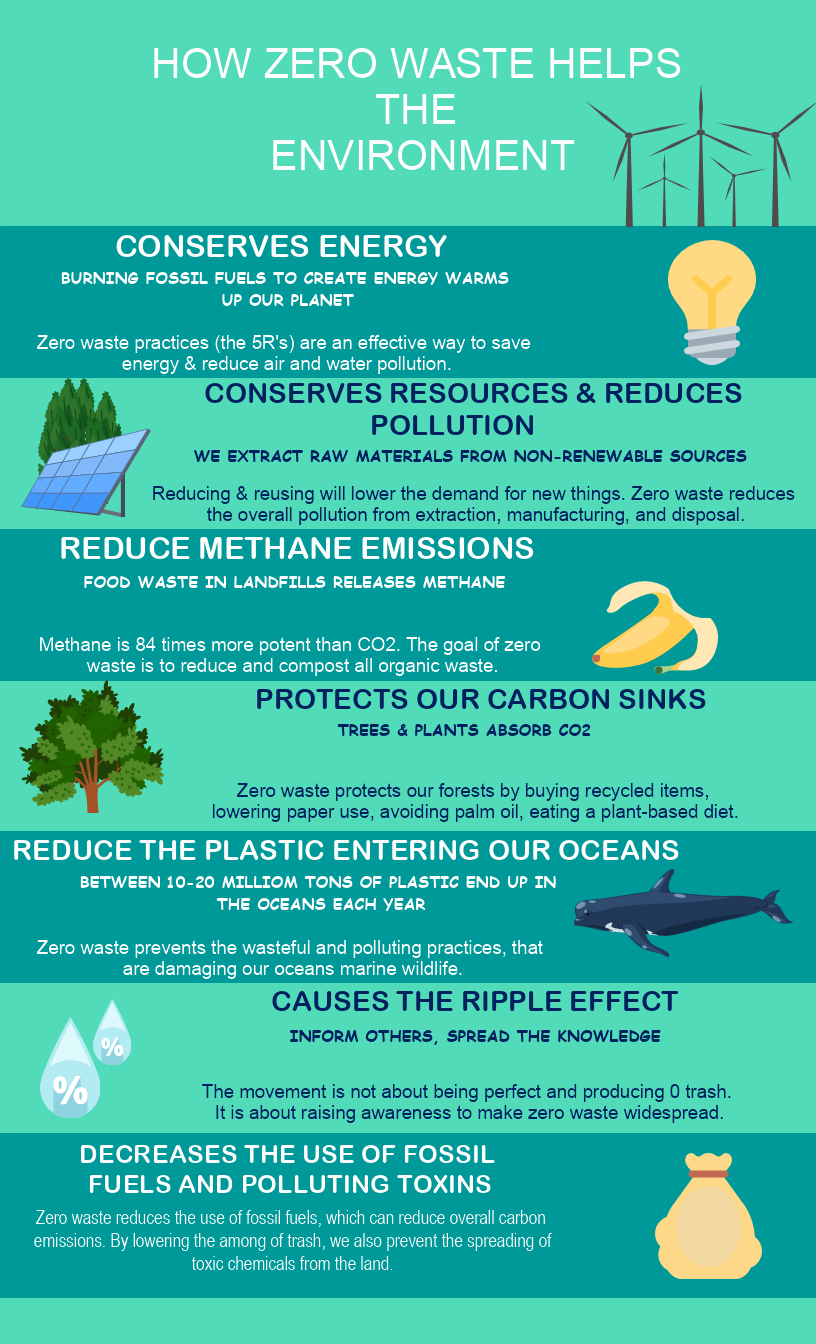This is a vertical rectangular poster illustrating how Zero Waste helps the environment, divided into nine horizontal sections. The topmost section, with an aquamarine background, features the title "HOW ZERO WASTE HELPS THE ENVIRONMENT" in white capital letters alongside images of wind turbines.

The following section, in teal, states "CONSERVES ENERGY" in white font, accompanied by a cartoon-style light bulb and explanatory text. The next section is in aquamarine with dark blue text that reads "CONSERVES RESOURCES AND REDUCES POLLUTION," featuring a solar panel among trees and explanatory details.

In teal again, "REDUCES METHANE EMISSIONS" is displayed with a cartoon banana peel, followed by another aquamarine section with "PROTECTS OUR CARBON SINKS" in dark blue text and an image of a large green tree.

Continuing in teal, the next section states "REDUCES THE PLASTICS ENTERING OUR OCEANS" with a cartoon whale image. The subsequent aquamarine section, featuring water droplets with percentage signs, reads "CAUSES THE RIPPLE EFFECT" in dark blue text.

Lastly, in teal, "DECREASES THE USE OF FOSSIL FUELS AND POLLUTING TOXINS" is displayed with explanatory text and a cartoon money bag, concluding with a thick aquamarine rectangle at the bottom of the poster.